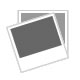In this indoor image, two old-timey dolls are seen sitting with their backs facing us on a round table adorned with a black, gray, and white checkerboard tablecloth. The background is solid black, making the dolls and their intricate details stand out. Both dolls are mounted on stands. The doll on the left is positioned on a white stand, and she is adorned with a straw hat, a black and white shawl, and a red skirt featuring a floral design with decorative stitching. Her white shirt peeks out from under her shawl. The doll on the right has a dark hair or a dark hat that blends seamlessly into the black background, topped with a light brown wicker basket. She is dressed in a green skirt with embroidered flower patterns along the bottom and wears a floral-colored long-sleeve shirt. Her left arm is raised slightly. Both skirts are voluminous, revealing their small brown wooden legs at the bottom of the image. The meticulous arrangement and detailed attire suggest a possibly Swiss theme in their clothing styles.